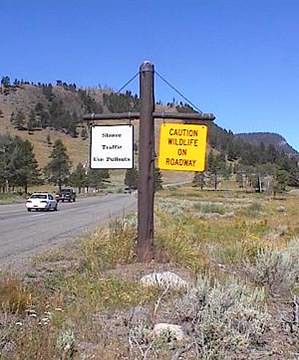The image depicts a slightly blurred, outdoor scene featuring a two-lane road with a white sedan heading away and a dark-colored truck (possibly blue or black) approaching. The road lies amidst foothills or low mountains, with scrubby trees, rocks, and patches of scrub brushes and yellowy flowers scattered around. In the foreground, there is a prominent T-shaped brown signpost with two signs: a bright yellow-orange one on the right stating "Caution: Wildlife on Roadway" in red, and a smaller, white sign on the left mentioning something about traffic, though its details are indistinct due to the image's poor quality. The sky is clear and blue, contributing to the serene, slightly nostalgic atmosphere reminiscent of a photo taken before the digital era.